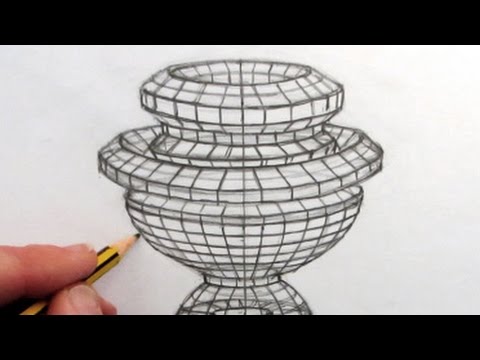This photograph captures a detailed pencil drawing in progress, held by a left-handed artist. The yellow and black striped pencil, grasped by the artist's three fingertips, is actively sketching on the white paper. The drawing is an abstract, multi-layered structure that strikingly resembles a vessel or trophy with a complex structure. The form has a small cylindrical base that broadens midway, creating a larger, grid-like bowl composed of interlocking square tiles, which then tapers into a flared top section. Atop this larger section sits another smaller bowl that once again tapers and then flares outward. In the background, two solid black bars, one at the top and one somewhere within the image, add a touch of visual contrast to the monochromatic sketch. The entire composition exudes an intricate blend of geometric patterns and abstract design, evoking an almost glass-like texture in its detailed, layered arrangement.